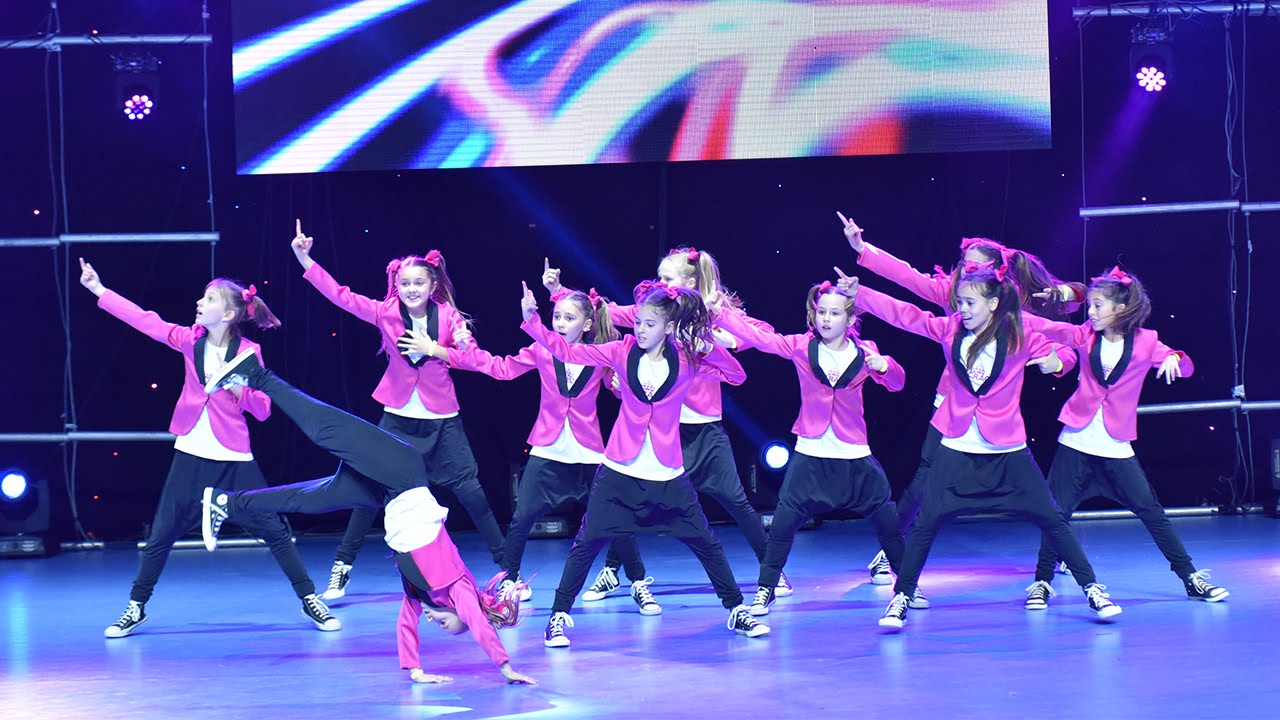In this vibrant image captured during a dance performance, we see a dynamic group of approximately ten young girls, likely aged 12 to 14, mid-routine on a well-lit stage. The dancers, all of whom appear to be Caucasian, are dressed in matching pink jackets over white shirts, paired with black pants and black and white Converse sneakers. The focal point is a girl at the front executing a cartwheel, while the others behind her strike a dab pose with their right arms extended and left arms bent. Their hair is adorned with pink ribbons, adding a unified and lively touch to their appearance.

High above them, a large screen displays a mesmerizing wave of colors that complement their outfits. The stage beneath them is a hard, reflective surface, casting hues of blue and purple from the vibrant stage lighting. The entire scene suggests a structured yet joyous performance, possibly part of a talent show or similar event, with the overall energy reflecting the girls' enthusiasm and enjoyment of their dance.